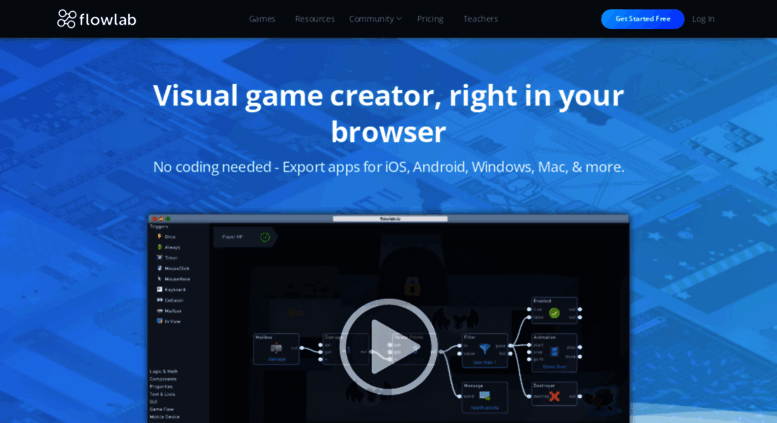This is the homepage of Flow Lab, a platform designed for creating games without any coding knowledge. At the top, there's a black navigation bar featuring the Flow Lab logo, which resembles a network of interconnected nodes. The navigation options include titles such as Games, Resources, Community, Pricing, and Teachers, with additional links for "Get Started for Free" or "Login" on the right side.

The main page has a serene blue background, evocative of a world-building simulation game, akin to SimCity, with various plots of land presented in a blue tint. Centrally placed is a clickable video that presumably provides an introduction to the platform and demonstrates its features. Prominently displayed is the tagline, "Visual game creator right in your browser. No coding needed. Export apps for iOS, Android, Windows, Mac, and more," suggesting the platform’s ease of use and versatility. The page also includes a detailed and professional-looking video and an embedded graphic, adding to the overall sophisticated presentation of the Flow Lab website.